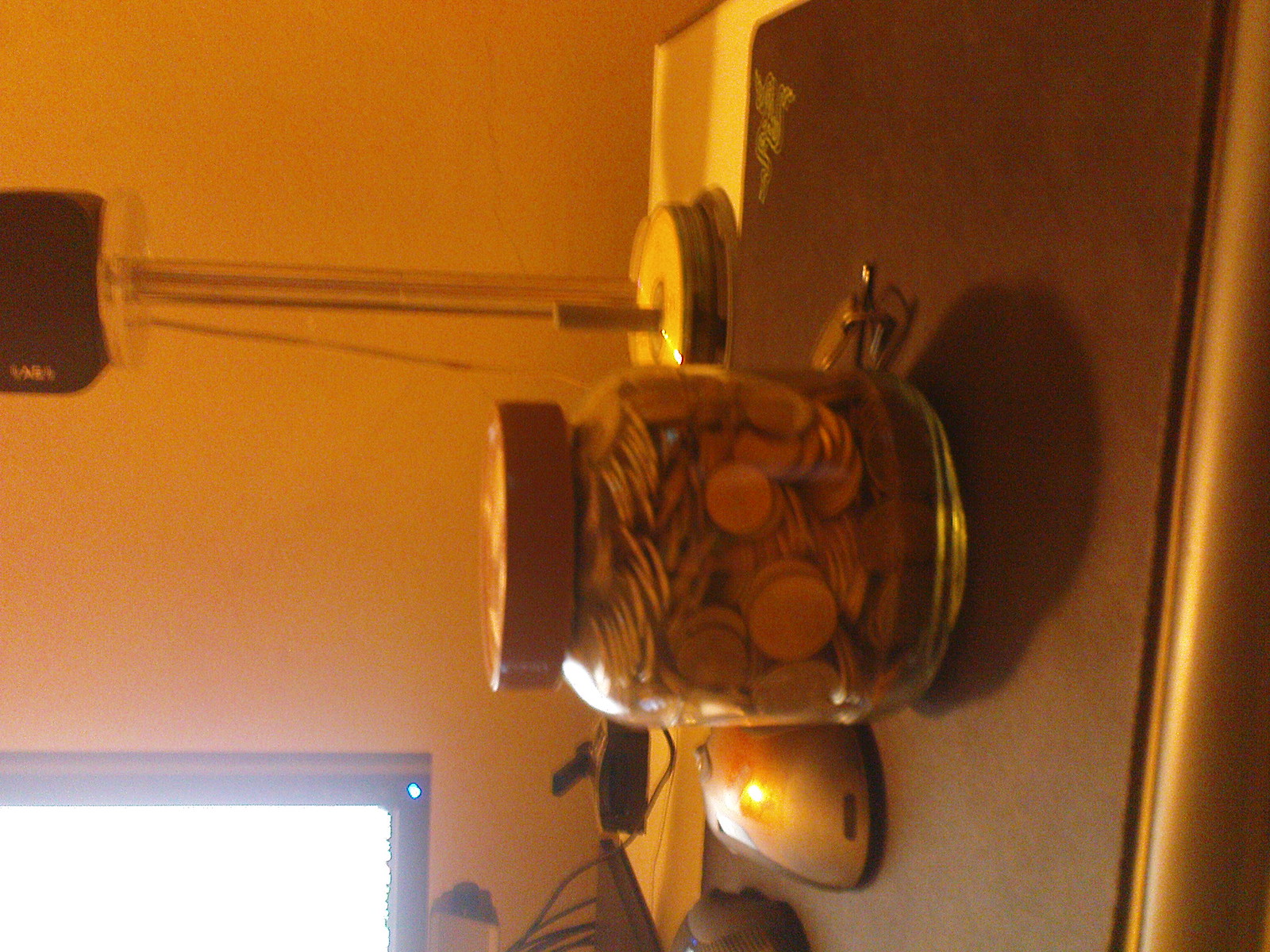The image is a grainy, low-quality, color photograph taken indoors with poor lighting that gives the entire scene an orange glow. The photo itself is turned sideways, requiring you to tilt your head to the left to see it properly. At the center of the image, there's a close-up of a glass jar with a brown twist-on lid filled with coins, predominantly silver, sitting in the middle of a white desk. To the right of the jar, there's a black mouse pad with a Razer logo, on which sits a silver computer mouse. To the left of the image, you can see part of a very bright computer monitor emitting significant glare. Also on the desk is a lamp located towards the back. There are some additional items around the jar, possibly a set of keys or a pair of glasses, but the orange tint and the bright screen make it difficult to discern finer details.